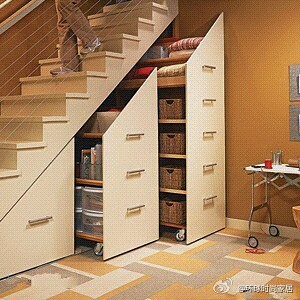The image depicts a well-organized storage solution under a white staircase within a home. Three roll-out cabinets are seamlessly integrated beneath the stair's structure, each featuring vertical edges to fit perfectly. The tallest cabinet at the back, opened the furthest, boasts five handles and six shelves, some of which hold brown boxes. In the center, a medium-sized drawer with three handles has three shelves, storing plastic containers. The bottom drawer, equipped with a single handle, remains closed. The stairs are protected by a string barrier that runs vertically, paralleling the steps. A person clad in brown khaki pants and sneakers is seen descending the staircase, visible only from the knees down. The floor showcases a patchwork of rectangular tiles in varying shades of light orange, brown, and cream. To the right, a mobile table with chrome legs, black wheels, and a white adjustable top stands against a light brown wall. The overall color palette includes brown, orange, tan, white, blue, red, gray, and black, creating a warm and inviting atmosphere.